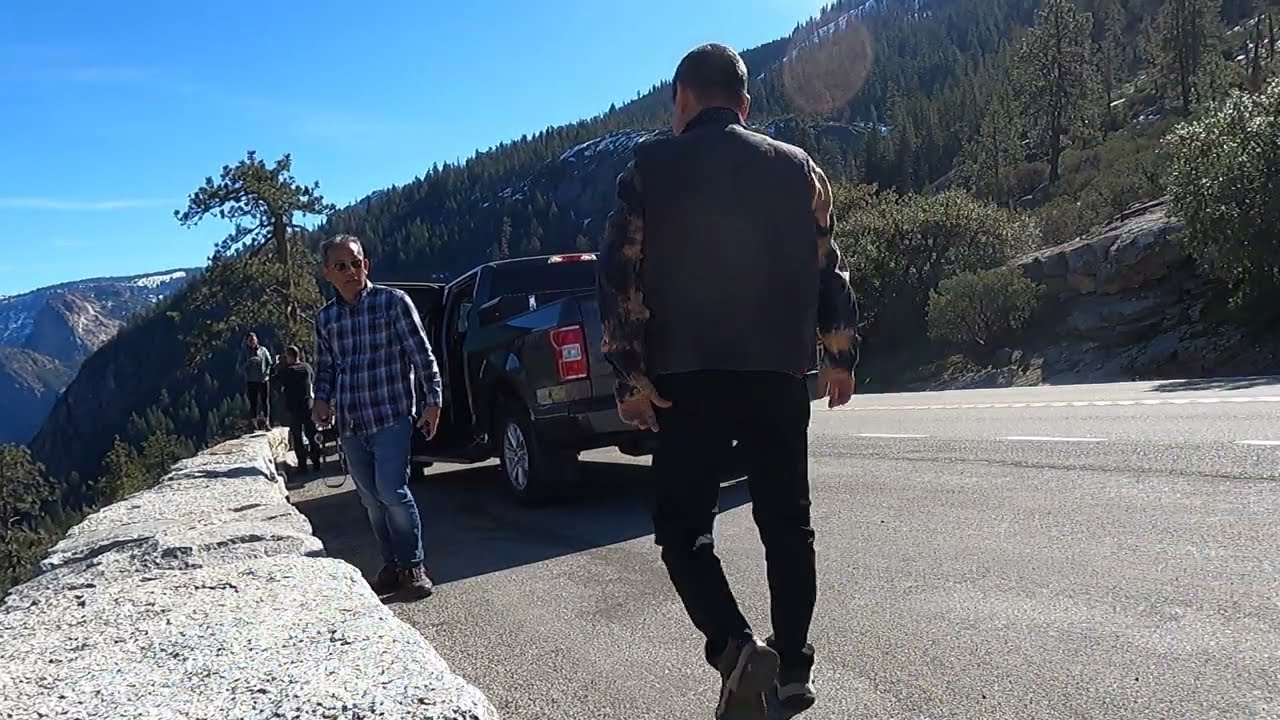The image captures a dynamic outdoor scene along a mountainside road, bustling with various people and a backdrop of picturesque natural elements. Dominating the foreground, a man with short hair wears a gray jacket, black pants, and sneakers, walking down the street. Walking towards him, with his back to the camera, is another man in a blue and white flannel shirt, blue jeans, and brown boots. In the far distance is a parked gray truck, near which a man, dressed in a long-sleeve shirt and black vest, navigates toward the vehicle. 

The scene is framed by lush greenery, with multiple hills and a mountain range covered in trees and dense vegetation. The road, marked with a dashed white line and a solid yellow line at its edges, curves around the hillside, enhancing the scenic backdrop. Among the landscape, a tall tree stands prominently beside the road. Additionally, on the left side of the road, a stone barrier marks the hill's edge where a woman stands on rocks, posing for a photo taken by a nearby man. The blue sky above is mostly clear, complementing the vibrant, outdoor atmosphere reminiscent of a popular tourist spot.